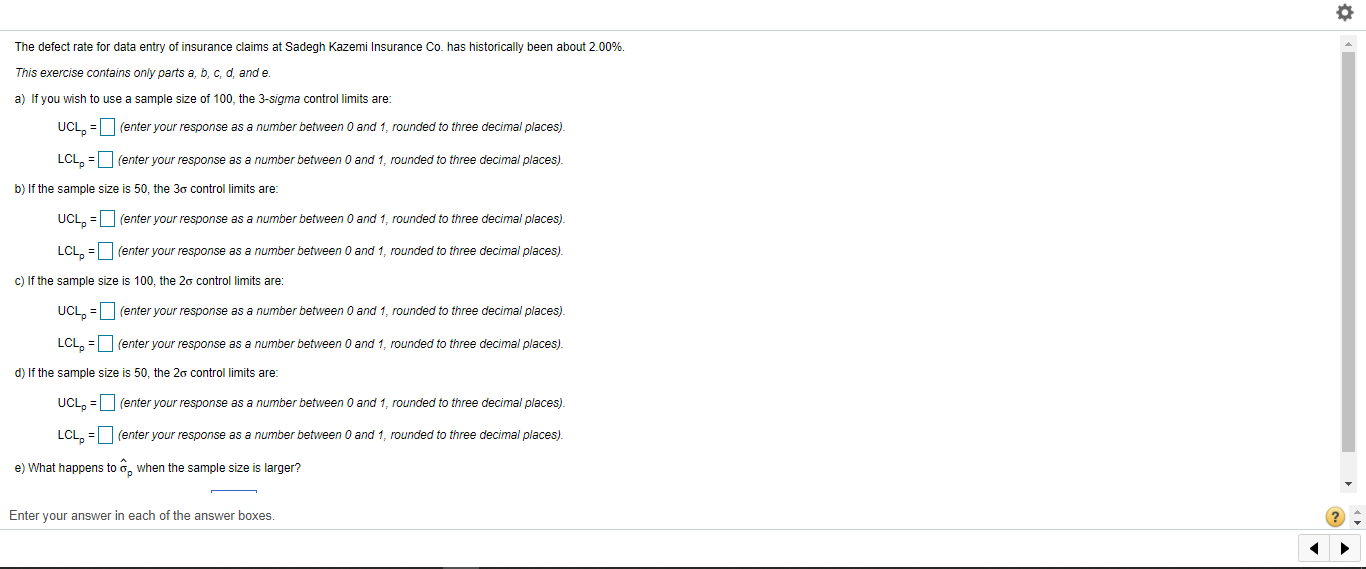Detailed Descriptive Caption:

The image features a predominantly white background with black text detailing an exercise related to insurance claims at Sadegh Kazem Insurance Corp. Key elements of the interface are annotated to provide visual cues and navigation options. At the top right, there is a grey settings icon shaped like a key. Below this, aligned on the right side, is a vertical slider for scrolling through the content. Located at the bottom right is a yellow question mark icon, likely providing additional help or information.

On the central left side of the image, the instructional text begins: "The Defect Rate for Data Entry of Insurance Claims at Sadegh Kazem Insurance Corp. has historically been about 2%." The exercise is divided into several parts, labeled A through E:

- **Part A:** "If you wish to use a sample size of 100, the 3 Sigma control limits are..." followed by two checkboxes labeled "UCLP" and "LCP". Users are instructed to enter their responses as a number between 0 and 1, rounded to 3 decimal places.
  
- **Part B:** "If the sample size is 50, the 3 Sigma control limits are..." Here, users enter the details for both "UCL" (Upper Control Limit) and "LCL" (Lower Control Limit), also rounded to 3 decimal places.
  
- **Part C:** "If the sample size is 100, the 2 Sigma control limits are..." again requesting values for "UCL" and "LCL".
  
- **Part D:** "If the sample size is 50, the 2 Sigma control limits are..." asking for "UCL" and "LCL" entries, concluding with, "What happens?"
  
- **Part E:** Ends with a question, "What happens to Sigma P when the sample size is large?"

At the bottom of the image, instructions specify to "enter your answer in each of the boxes." These input boxes are colored blue, designated for both UCL and LCL values. Additionally, two navigational buttons exist to allow movement to the left and right, though their exact locations are not specified in the voice description.